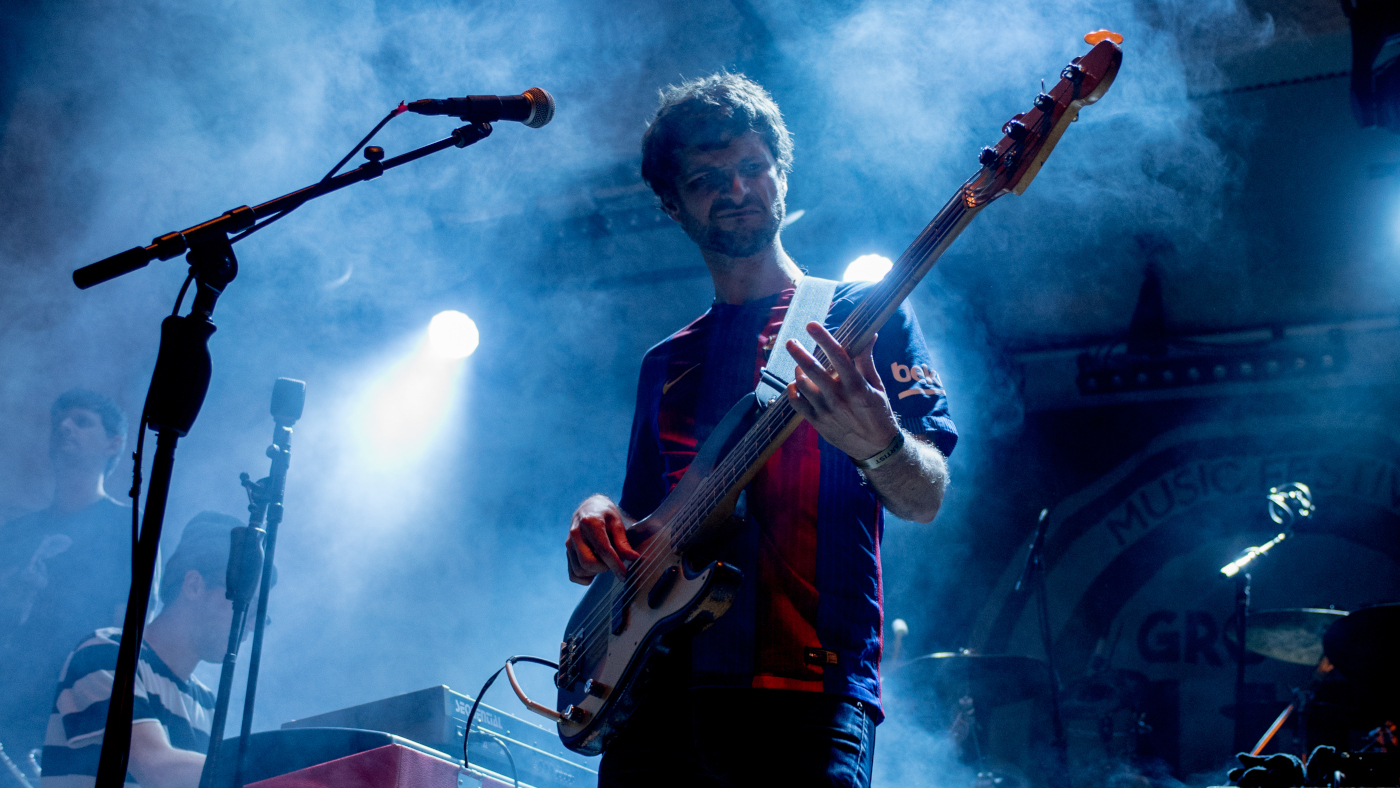The image captures a dynamic live performance, featuring a white-skinned man with a thick head of brown hair and a beard, fervently playing a brownish-gold bass guitar. He’s decked out in a blue and red football jersey, resembling a Barcelona kit, with Nike and yellow details, paired with jeans. His face scrunched in concentration, he skillfully manipulates the bass with his right fingers while his left hand hovers over the bridge. The stage is enveloped in an atmospheric haze created by fog, with stage lights cutting through, lending a dramatic flair to the scene. A microphone on a stand with an extender is positioned to his left.

Behind him, a man clad in a black and white horizontally striped shirt and glasses is seated at a keyboard, illuminated by overhead lights. Further back, another individual can be seen gazing towards the audience, adding depth to the scene. The backdrop prominently features a large sign reading “Bearly Music Festival,” enhancing the festivity's context. Musical equipment, including a drum set, is subtly visible in the background amidst the stage fog, encapsulating the electric ambiance of the live performance.